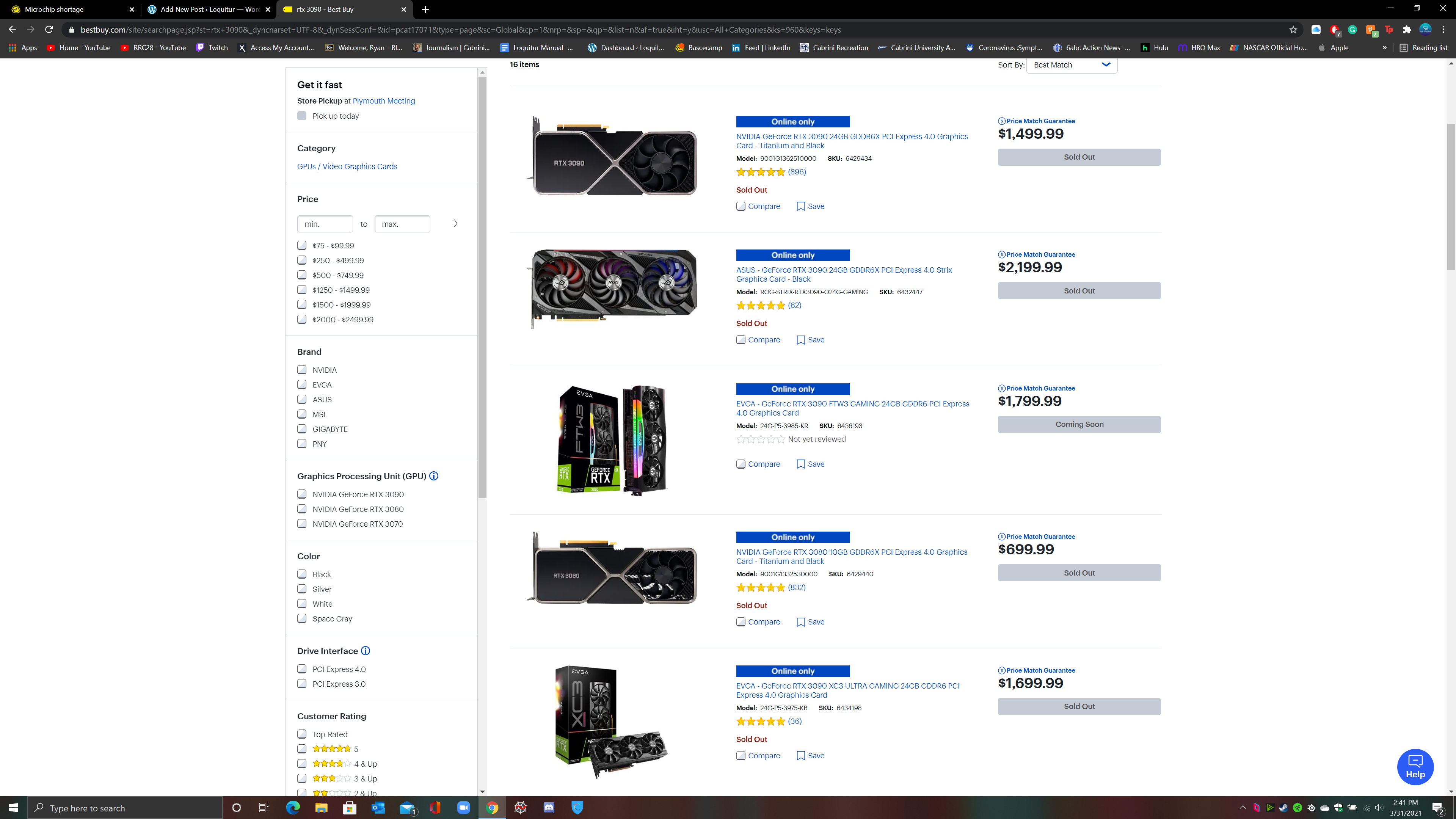In the image, a web browser window with three tabs open is displayed. The first tab is dedicated to information about the "microchip shortage." The second tab is showcasing the "Add New Post" page in WordPress, indicating a content management activity. The third tab is the BestBuy website, specifically showing a search for RTX 3090 graphics cards. 

In the search results, five graphics cards are listed, including four RTX 3090 models and one RTX 3080 model. The prices for the RTX 3090 cards vary, with listed amounts of $699.99, $1,799.99, $2,199.99, and $1,499.99. In the top right corner of the browser window, standard window control buttons for minimizing, adjusting the size, and closing the window are visible. 

Several browser extensions are also displayed, including an ad blocker and a prompt to add more extensions. At the bottom of the screen, the taskbar features various icons, including Microsoft Edge, File Explorer, Windows Store, Outlook, Microsoft Office suite, Google Chrome browser, and Discord.

The image overall highlights a context of multi-tasking online activities, featuring research, content creation, and online shopping.